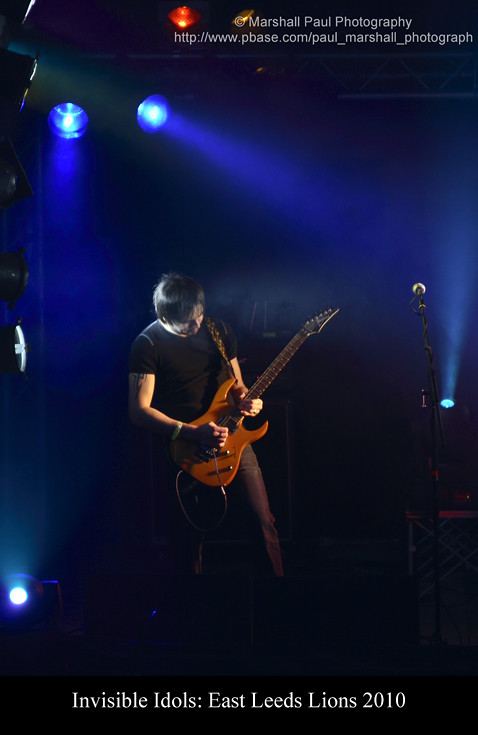The image captures an intense moment of a guitarist performing on stage, characterized by dark, atmospheric lighting dominated by blue and black hues. Four vivid blue spotlights illuminate the scene, framing the singular figure of the musician, who has short black hair and is dressed in a black shirt and indeterminate colored pants, potentially gray or brown due to the shadows. His right arm features a dark tattoo, partly obscured by the dramatic lighting. He dons a bracelet or wristband, adding to his rocker persona. The guitar he plays is a striking orange hue, held confidently at the lower fretboard. The guitar strap sports a striking design, possibly yellow or orange flames on a black background. Nearby, a microphone on a stand waits to the right, though he doesn’t appear to be using it. At the bottom of the image, white text reads “Invisible Idols; East Leeds Lions, 2010.” In the top right corner, more text credits the image to "Marshall Paul Photography" along with a website link. The scene conveys a moment of musical focus and artistry, emphasizing the guitarist’s solitary presence on stage.